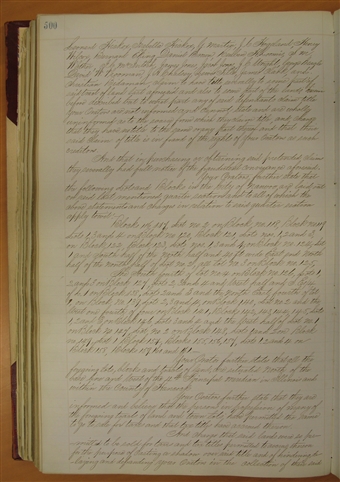The image depicts an aged page from a substantial journal or ledger, set atop a brown wooden table. The photo is taken from a top-down view, providing a clear perspective of the open book. The pages are yellowed with age, hinting at the document's antiquity. Handwritten in old-style cursive script, the ink appears either black or light gray, slightly slanted to the right, indicative of a right-handed writer. At the top left corner of the exposed page, the number "500" is marked in blue ink. The page contains seven distinct paragraphs of difficult-to-read English text, meticulously written by hand. Other pages of the book can be seen layered beneath, and the book itself has a dark red and white cover. The cursive writing and the aged, yellowed paper suggest the text was created before the advent of typewriters, capturing a slice of history in its original form.